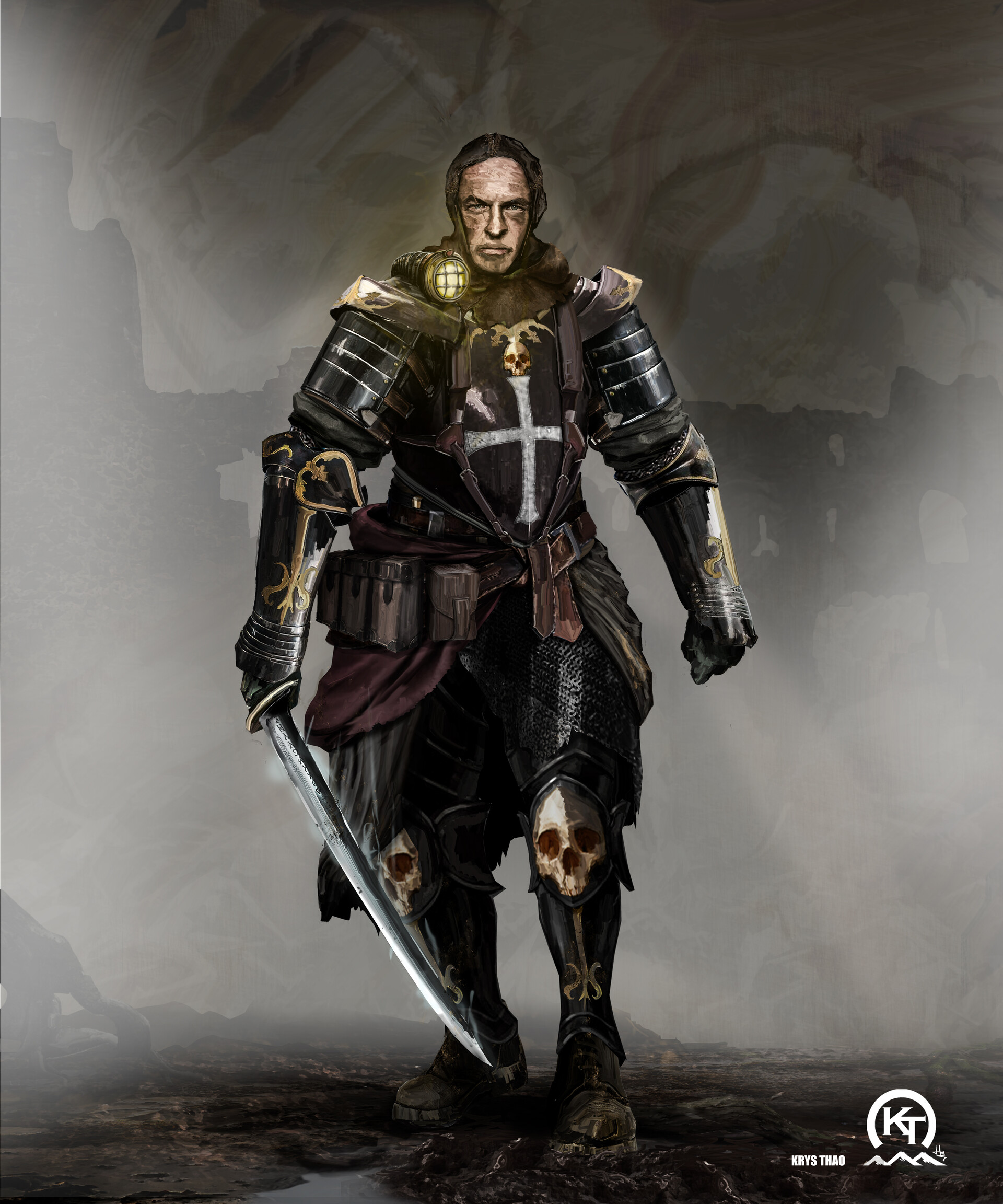This detailed image appears to be a computer-generated or AI-created piece, possibly concept art or a stylized painting. The focal point of the image is a stern, white male warrior clad in heavy black armor accented with white and gold details, including gold skulls and intricate designs. His armor covers his shoulders, forearms, wrists, thighs, and shins, featuring knee guards painted with skull faces. He wears a helmet that obscures his hair and a protective cape that is tied around his waist. The warrior has a silver cross emblazoned on his chest, above which a skull is depicted, and a small green light is attached below his neck. 

In his left hand, he holds a large silver sword pointed downward from left to right. His expression is angry as he gazes directly at the viewer. The background is misty and foggy, with hints of broken structures, rocky surfaces, hills or mountains, and streams of water, complemented by a gray sky with white beams streaming down. 

In the bottom right-hand corner of the image, there is a logo featuring three mountainous peaks beneath a semicircle, accompanied by the initials "KT" and the name "Chris Thao" or "Christ's Help."